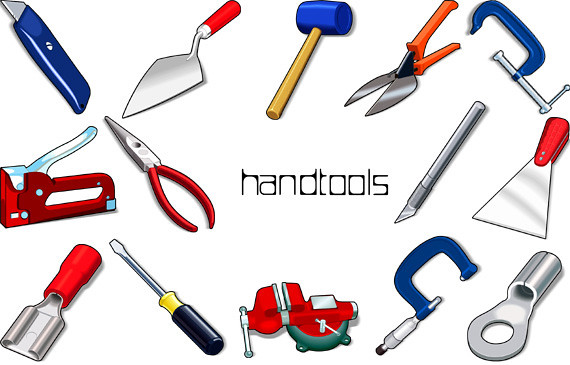The image features a collection of cartoonish-styled hand tools displayed on a white background. At the center of the image, the words "hand tools" are highlighted. The tools, arranged in a circular pattern around the text, include:

- A blue X-Acto knife (box cutter) situated in the upper left corner.
- A red-handled trowel next to the X-Acto knife.
- A blue-headed rubber mallet.
- An orange-handled pair of snips (shears).
- A blue c-clamp located in the upper right corner, with another blue c-clamp nearby.
- A flathead screwdriver with a yellow and black handle.
- Multiple electrical connectors, with one prominently red.
- A red power stapler.
- A pair of red needle-nose pliers above the stapler.
- A red-handled razor blade holder near the bottom left.
- A red vise with a silver and green base located towards the lower left.

The overall arrangement and colorful, exaggerated details suggest the image may be used as symbols or educational illustrations for identifying various hand tools.